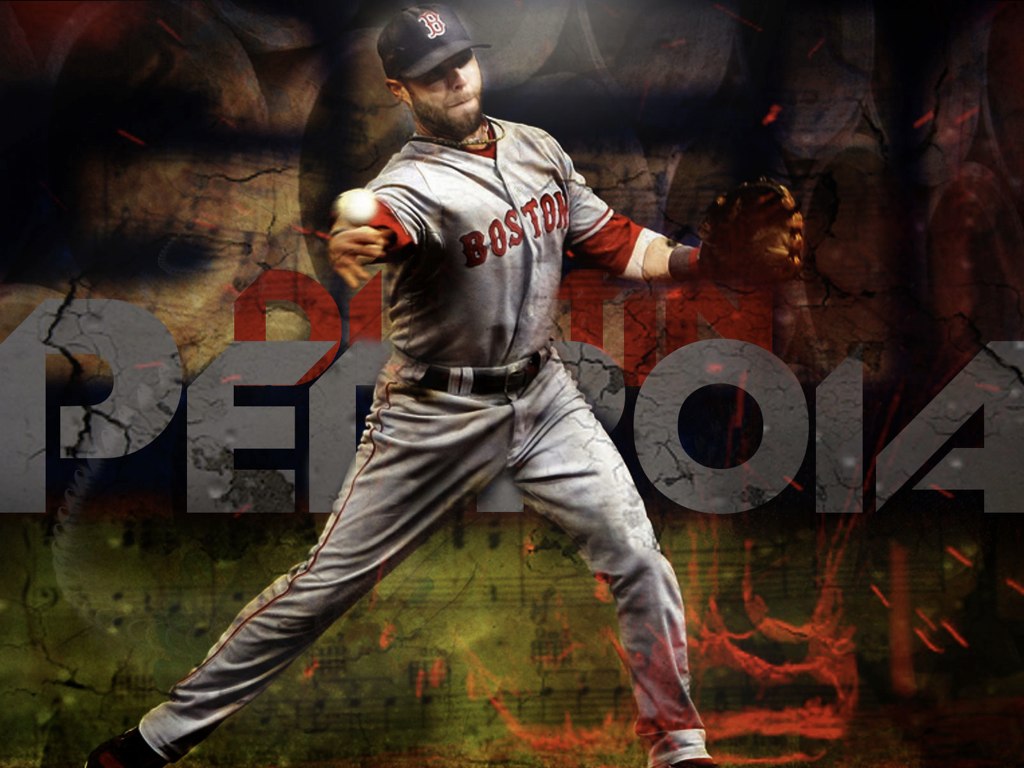The image captures a Boston baseball player at the center, framed in an action pose. He's wearing a gray shirt with red accents and the word "Boston" in red on the front. The shirt is paired with light gray pants, a black belt, dark shoes, and a dark blue cap featuring a red "B" outlined in white. The player is bearded, sporting a mustache, and wearing a necklace. 

His right hand is extended forward, having just thrown a ball that is still visible near his hand, while his left hand, wearing a brown glove, is also stretched out. His stance is wide with legs far apart, suggesting a moment of dynamic motion. 

The backdrop consists of a colorful wall that resembles graffiti or a graphical artwork, blending colors like green, red, gray, and black, with hints of musical sheet textures. There are visible letters in gray, starting from left to right: P, E, and then O, I, A on the other side. The blurred and abstract nature of the background adds to the vivid portrayal of the scene.